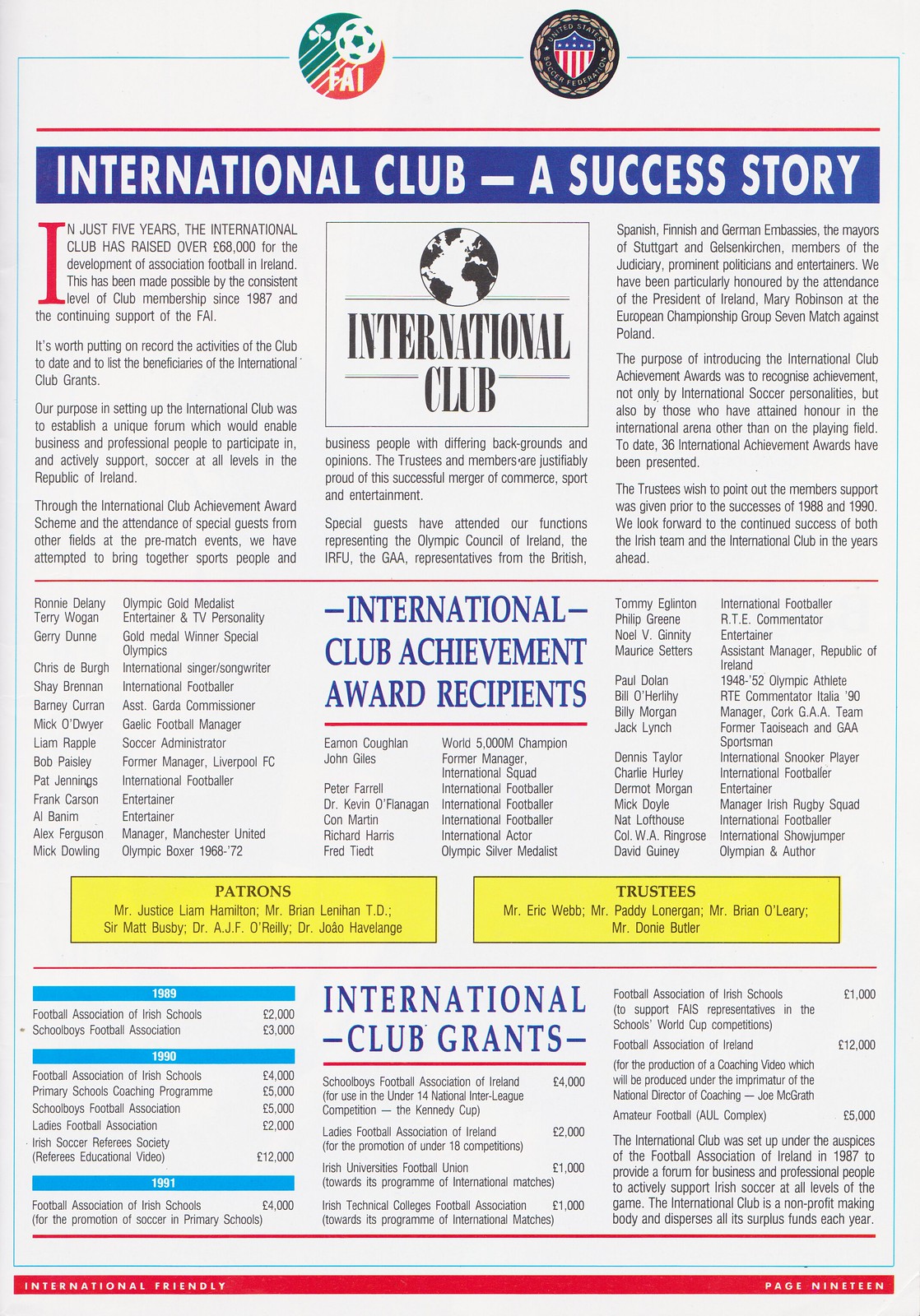This is a detailed photographic scan of a magazine page dedicated to the International Club, showcasing its achievements and organizational details. The page features a white background with several design elements for emphasis. At the top left, there are two symbols: a green and red circle showing a soccer ball and a circle resembling an official seal. The headline beneath these symbols reads "International Club: A Success Story," accompanied by a black and white image of the world. 

The main article commemorates the club’s efforts since its establishment in 1987 under the Football Association of Ireland (FAI). It lauds the club for having raised over £68,000 in five years to support Irish soccer and for hosting various notable guests from the worlds of sports, politics, and entertainment, including the President of Ireland, Mary Robinson.

The page is divided into three main sections. The first section comprises three columns elaborating on the club's origins, purpose, and milestone achievements. A prominent red line runs horizontally to separate this part from the next.

The second section is titled "International Club Achievement Award Recipients" in blue all-capital letters. It lists notable awardees such as Olympic gold medalist Ryan Delaney, entertainer Terry Wogan, and former Liverpool FC manager Bob Paisley. Flanking this list are two yellow rectangles labeled "Patrons" and "Trustees," detailing key supporters of the club.

The final section, titled "International Club Grants" in blue capital letters, outlines financial contributions made by the club to various football associations and educational programs from 1989 to 1991. Each year is itemized with corresponding amounts and purposes, such as £12,000 for a referees' educational video in 1990.

A red border at the bottom includes the note "International Friendly Page 19" as a navigation aid. 

This comprehensive depiction represents the International Club's holistic engagement with sports, community, and cross-border relations.